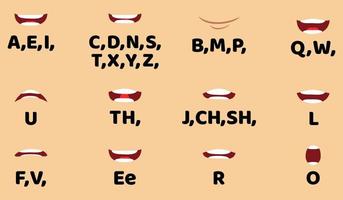This detailed chart illustrates various mouth positions associated with the pronunciation of specific letters. 

- In the top-left corner, an AEI-labeled mouth shows an almost smiling position, with the top and bottom teeth separated by a small gap.
- Adjacent to it, a mouth labeled CDNS TXYZ is also in a smiling position, but with the teeth separated by a very thin margin.
- The BMP-labeled mouth immediately after shows closed lips pressed together, forming a thin line.
- The next mouth, labeled QW, presents a wide-open smile with a significant gap between the top and bottom teeth.

The following row includes:
- A downturned mouth with visible top teeth, labeled U.
- A mouth in a neutral position with teeth moderately spaced, labeled TH.
- Another neutral-position mouth with slightly closer teeth, labeled JJ.
- A smiling mouth with medium-spaced teeth, labeled L.

In the final row:
- A somewhat downturned mouth with teeth relatively close, labeled FV.
- An upturned mouth with teeth spaced at a medium distance, labeled E.
- A neutral-position mouth with teeth a little close together, labeled R.
- Lastly, a wide-open mouth with significantly separated teeth, labeled O.

Each depiction offers a clear visual representation of the corresponding mouth shapes required for accurate articulation of these letters.